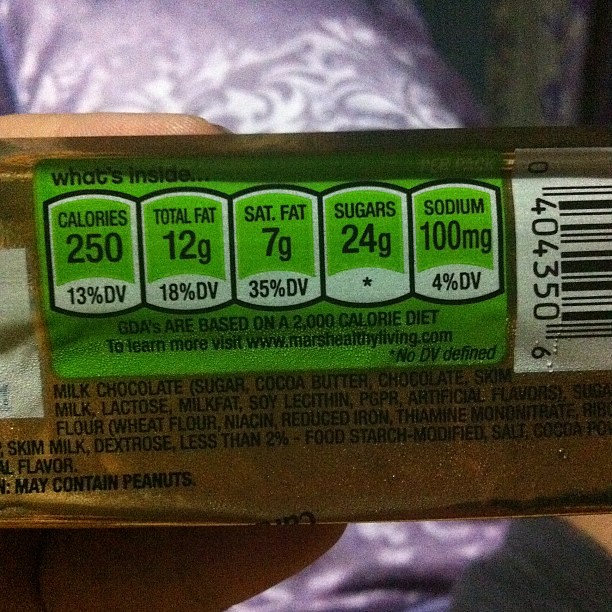The image features a close-up of someone holding a chocolate bar still in its gold foil wrapper, presumably a Twix bar, evidenced by the color and layout. The person's left hand is visible on the left side, gripping the wrapper with a thumb cut off by the frame and fingers partially behind the package. The detailed nutritional facts indicate the bar contains 250 calories, with 12 grams of total fat (18% DV), 7 grams of saturated fat (35% DV), 24 grams of sugars, and 100 milligrams of sodium (4% DV). A greenish rectangle on the wrapper lists multiple ingredients, including milk chocolate, sugar, cocoa butter, chocolate, skim milk, lactose, milk fat, soy lecithin, PG, PR, artificial flavors, wheat flour, niacin, reduced iron, thiamine, dextrose, modified food starch, salt, and cocoa powder. There's also a warning that it may contain peanuts. In the background, a purple cloth with white swirls is visible, possibly part of a bedspread. The person's leg in grey shorts can be partially seen at the bottom right of the image. The photo also includes a barcode on the right side and a white box on the left side of the wrapper.